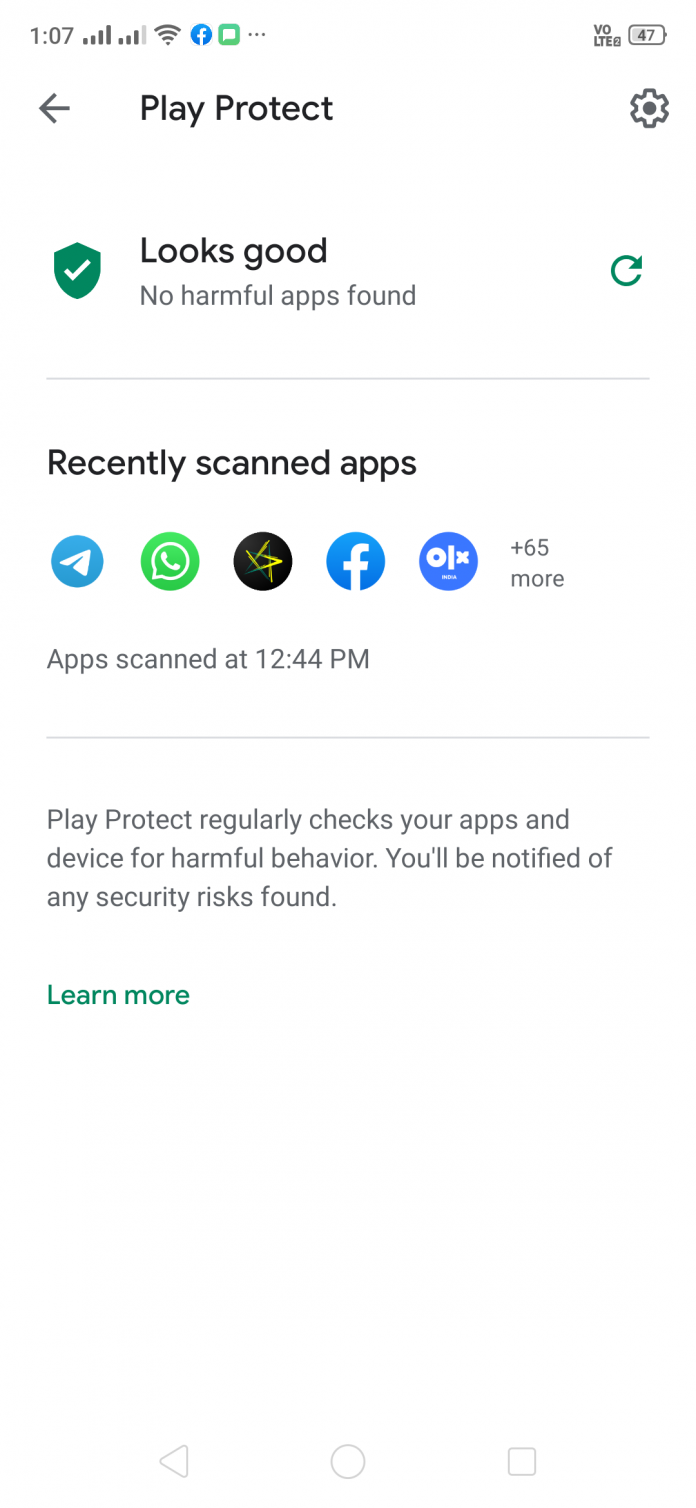Here is a cleaned-up and detailed caption for the image:

---

**A Mobile Phone Screenshot Detailing System Information and Security Status**

The screenshot, captured from a mobile phone, displays various status indicators and notifications on the device's screen. 

- **Top Information Bar:**
  - **Battery Life:** Displaying 47% remaining.
  - **Signal Strength Indicators:** Three bars representing different signal strengths, with the first bar full, the second bar nearly full, and the third bar empty.
  - **Wi-Fi Indicator:** Showing a strong, full signal.
  - **Icons:** Including a Facebook icon and an icon featuring three dots, likely representing additional options or notifications.

- **Main Notification Panel:**
  - **Left Arrow Icon with accompanying text:** "Play Project."
  - **Cog Icon:** Indicating a settings menu.
  - **Text Notification:** Reading "Looks good, no harmful apps found."
  - **Circular Arrow Icon:** Signifying a refresh or update command.
  - **Underneath the Circular Arrow Text:** "Recently scanned apps" with five visible app icons, including Telegram, WhatsApp, and Facebook. One icon is unidentifiable.
  - **Additional Scanned Apps Notification:** "+65 more apps scanned at 12:44 PM."
  - **Security Notification:** "Play Project regularly checks your app and devices for harmful behavior. You'll be notified of any security risk found."

- **Instructions and Further Information:**
  - **Learn More Link:** Highlighted in green, offering users additional information about the security checks.

---

This detailed description provides a comprehensive understanding of the different elements and notifications displayed in the screenshot.